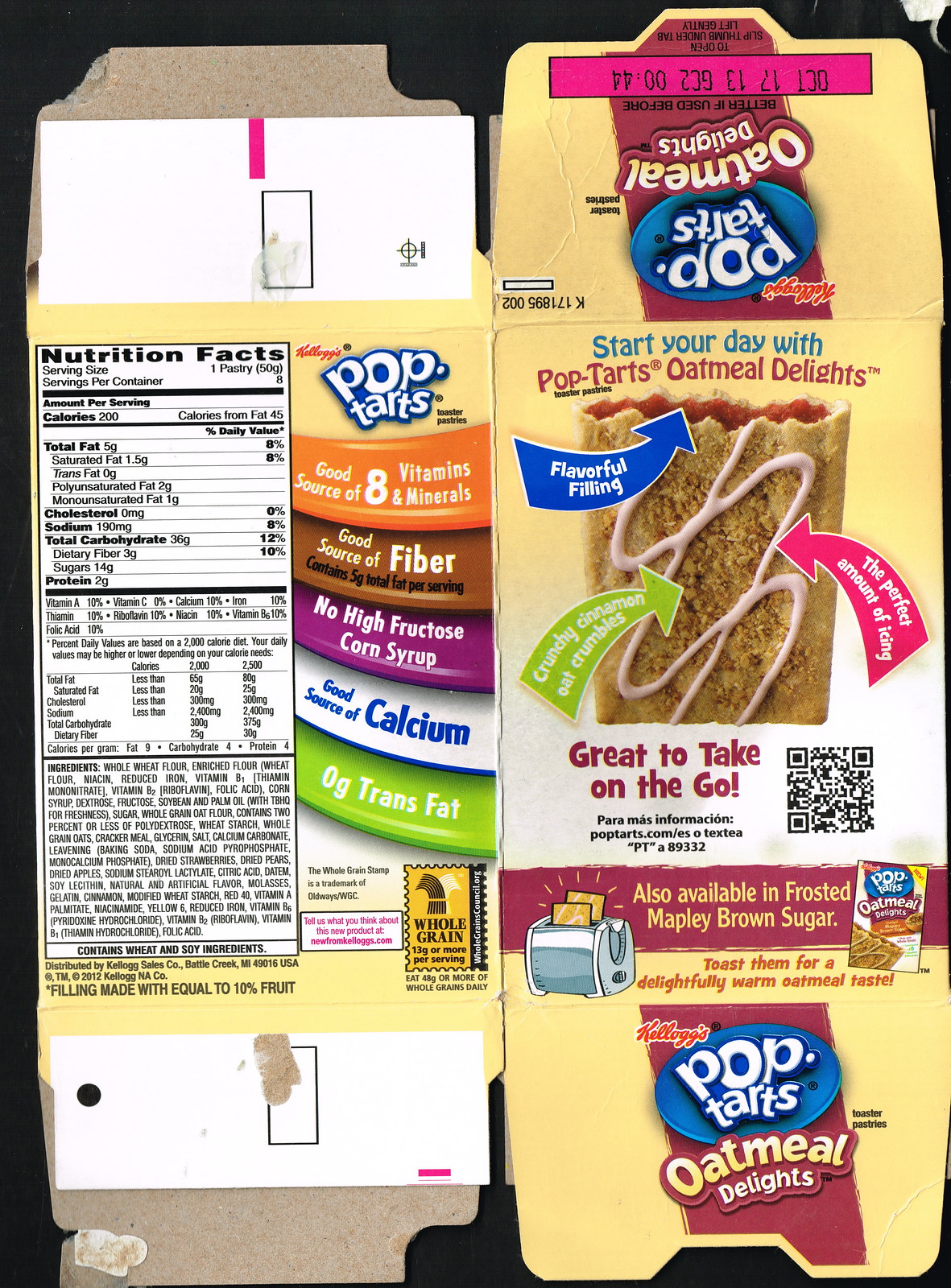The image showcases a flattened and unglued Kellogg's Pop-Tarts Oatmeal Delights box, fully spread out to reveal extensive details on both the front and side panels. The front panel prominently advertises the product with slogans like "Start your day with Pop-Tarts Oatmeal Delights," highlighting "flavorful filling, crunchy cinnamon oat crumbles, the perfect amount of icing," and noting that it's "great to take on the go." 

The box also features a QR code for additional information and text in either Spanish or Portuguese directing consumers to a website or a text number. The use-by date indicated on the box is October 17, 2013. 

The left-hand side of the box contains detailed nutritional facts, stating it as a good source of eight vitamins and minerals, fiber, and calcium. It boasts no high fructose corn syrup and zero grams of trans fat, with a breakdown of the calories, fats, carbohydrates, dietary fiber, sugars, and proteins per serving. The right-hand side mirrors these details, and the bottom of the box repeats the branding – "Pop-Tarts Oatmeal Delights."

Overall, the package is yellow with white accents and displays images of the toaster pastries with icing and red filling, conveying its enticing appeal and nutritional benefits comprehensively.